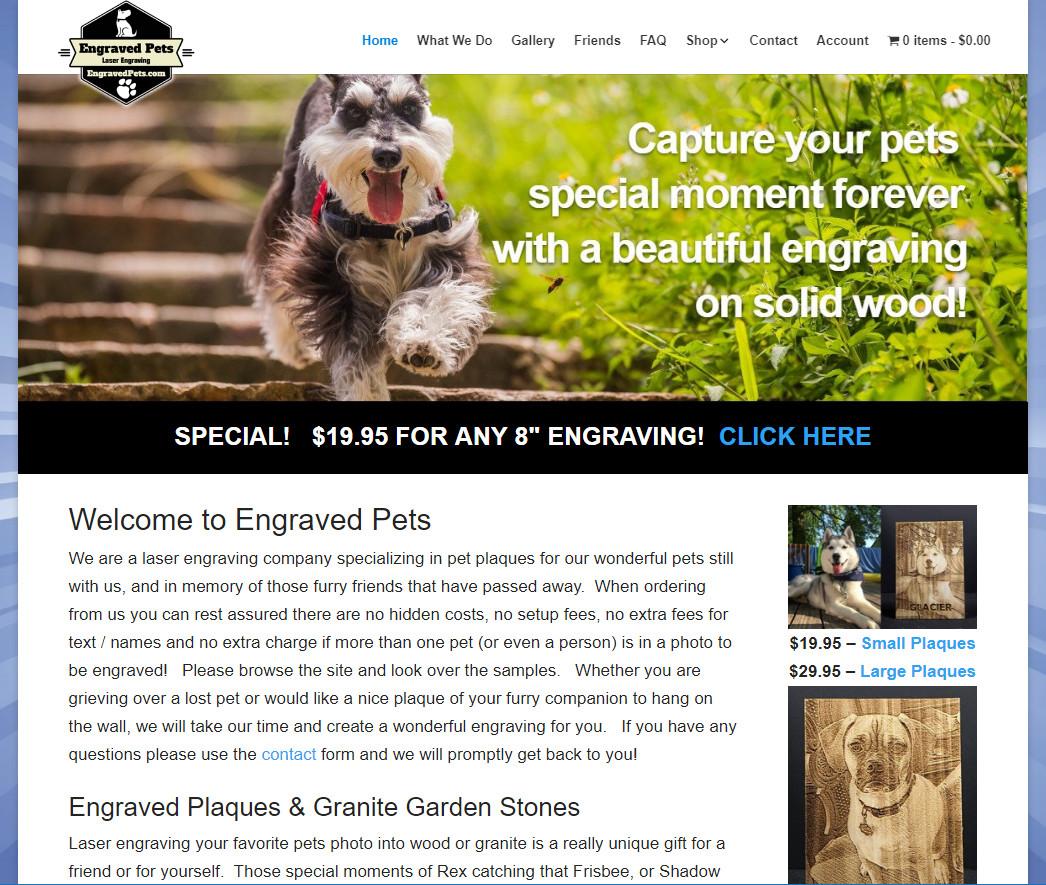This screenshot captures the homepage of the website "Engraved Pets Laser Engraving," found at engravedpets.com. The website's navigation menu, located at the top, includes several clickable options: Home, What We Do, Gallery, Friends, FAQ, Shop, Contact, and Account. Currently, the Home section is selected. The website indicates that there are zero items in the shopping cart, with a total balance of $0.00. 

The central headline reads, "Capture your pet's special moment forever with a beautiful engraving on solid wood," followed by a special offer: "Special $19.95 for any 8-inch engraving." A clickable prompt, "Click here," which is highlighted in blue text similar to the Home menu option, directs users to take action.

Further down the page, there is a visual comparison showing a photograph of a dog lounging on a patio and its corresponding wood engraving. Pricing details are provided: small plaques are priced at $19.95, while large plaques are available for $29.95.